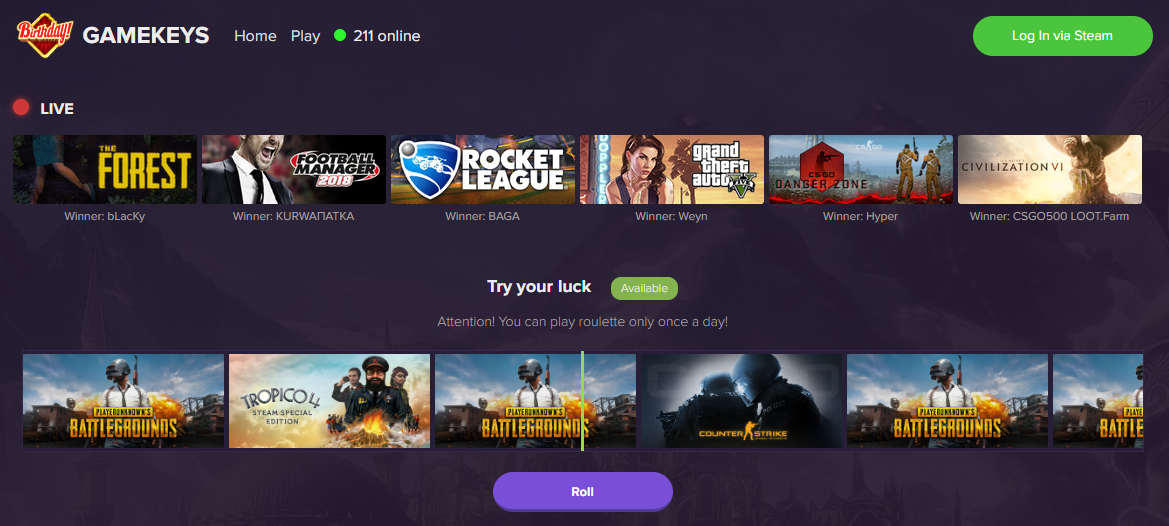The screenshot features a predominantly black background. In the upper left corner, a vivid red diamond outlined in yellow contains the word "BIRTHDAY" also in red and outlined in yellow. Adjacent to this, in all-white capital letters, reads "GAME KEYS." Further right, "HOME PLAY" is displayed in white text. Next to it, a fluorescent green circle features the text "2-1-1 ONLINE" to its right.

On the far right, there's a green oval button with "LOG IN VIA STEAM" written inside in white text. Approximately three lines down on the left side, a red circle appears next to the word "LIVE" in all-white capital letters. Below this, a series of rectangles follow, each containing an image and a name in white text underneath. The first rectangle features "Warner Blackie," followed by "Winner Bogoff" in the next.

Centered in the middle of the image, two lines down from the rectangles, is the phrase "TRY YOUR LUCK" in white text. To the right side of this phrase is a green oval button labeled "AVAILABLE." Two lines below that text, in gray letters, is a cautionary message: "Attention! You can play roulette only once a day!"

Further down, there's another row with various images, predominantly related to battlegrounds. At the bottom center of the screenshot, a purple oval button is labeled "ROLL."